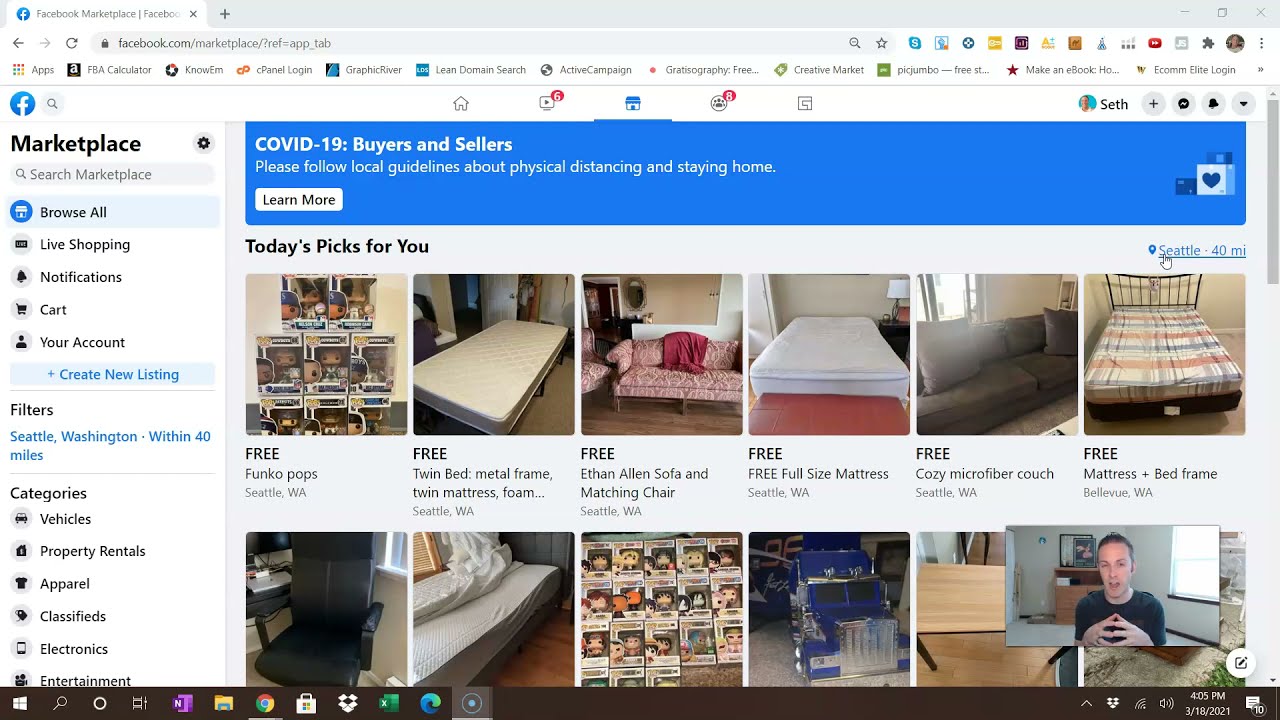This image captures a detailed view of an online marketplace interface, prominently highlighting a COVID-19 advisory at the top within a blue square. The advisory urges users to adhere to local guidelines regarding physical distancing and staying at home, accompanied by a white "Learn More" button. Below, the section titled "Today's Picks for You" showcases several free items available in Seattle, Washington, and Bellevue, Washington, including:

- Free Funko Pops
- Free Twin Bed Metal Frame with Twin Mattress Foam
- Free Ethan Allen Sofa and Matching Chairs
- Free Full Size Mattress
- Free Cozy Microfiber Couch
- Free Mattress and Bed Frame (Bellevue, Washington)

The visual section beneath features images of various items including a black desk chair, a mattress, Funko Pops figurines, a blue truck, and a brown stand or entertainment center. Additionally, a man in a black shirt is depicted with his fingers touching each other in one of the photos. On the left side of the screen, navigation options are listed, including "Browse All," "Live Shopping," "Notifications," "Cart," and "Your Account," along with various category listings.